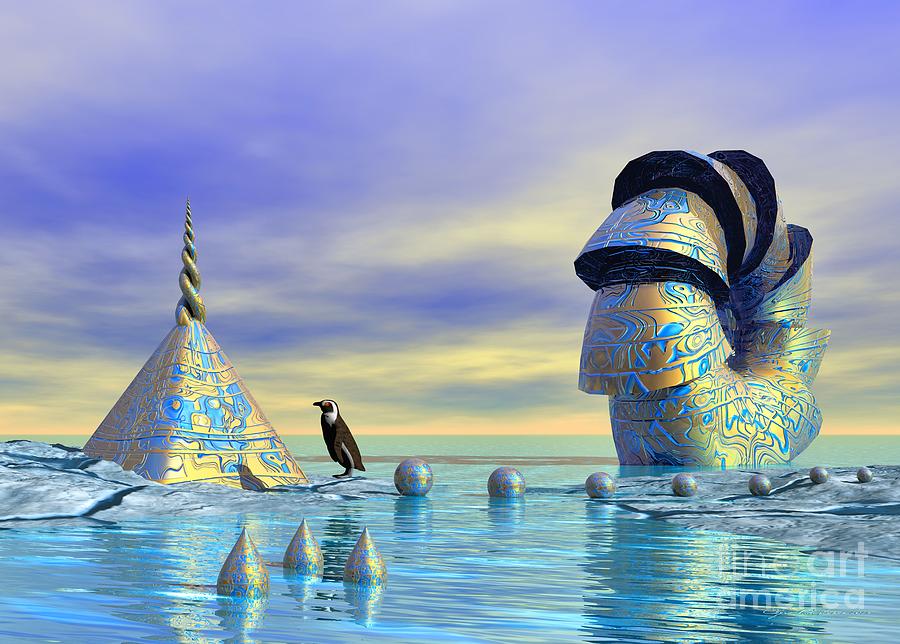This computer-generated image, possibly created by AI, presents a surreal and vibrant arctic seascape under a cloudy sky illuminated with gold and blue hues. The scene features intriguing ice-bound, metallic structures with a consistent blue and gold design that almost resembles hieroglyphs. To the left, we see a striking pyramid-like structure with two tapering shafts coiling around each other and culminating in a horn at the top. A small penguin, white and black with a red eye, stands adjacent to this pyramid, intently observing it. Rising from the water in the foreground, three cone-like structures mirror the metallic motif. In the center of the image, seven orbs of increasing size continue the blue and gold pattern, leading towards a layered, donut-shaped ring on the far right. These partial cones, forming the ring, suggest a donut shape crafted from a gold, metallic substance intricately modeled with ribbons of blue. The entire composition is underlaid with a watermark, "Fine Art America," subtly visible in the bottom right corner, marking it as part of an experimental and detailed digital art project.